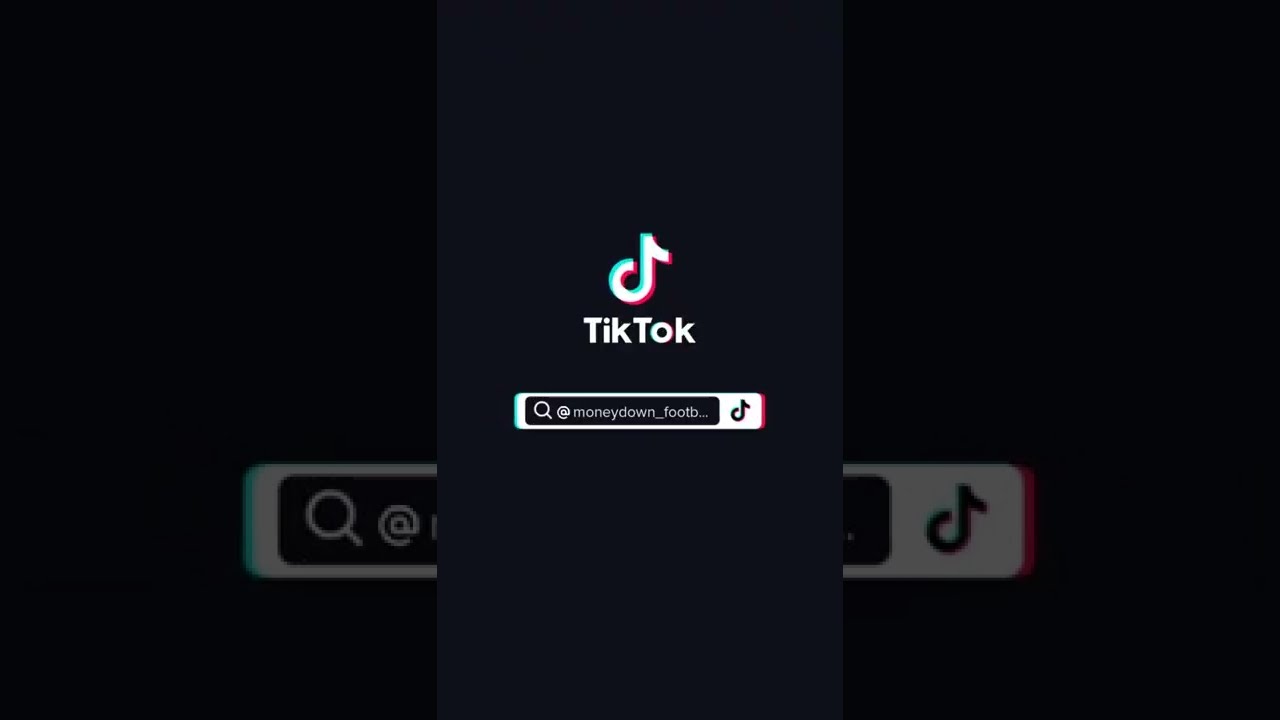The image appears to be a screenshot of the closing screen of a TikTok video. The background is entirely black, with a prominent white TikTok logo at the top resembling a musical note, accompanied by the text "TikTok" underneath. Below this logo and text, there's a search bar displaying the text "at money down underscore foot B...," likely indicating a username related to football. To the right of the search bar, another TikTok symbol is present. This central image is overlaid and framed by zoomed-in fragments of itself, creating a portrait-style photo effect commonly seen on cell phones. The entire composition is encased in mostly black rectangles, emphasizing the main elements against the dark background.